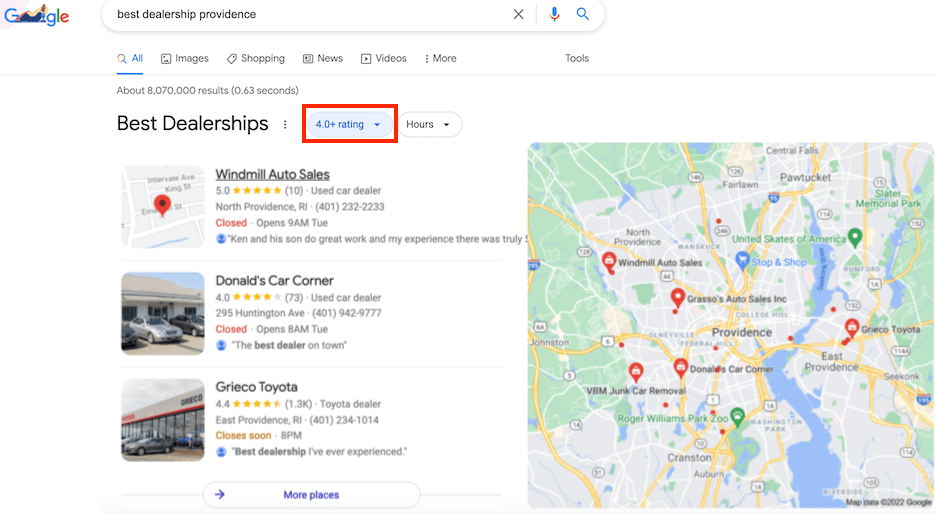The image is a screenshot of a Google search results page. In the top left corner, the recognizable Google logo in blue, red, yellow, and green hues is visible. Adjacent to the logo is the search bar, displaying the query "Best Dealership Providence." Below this bar, a navigation menu offers options such as All, Images, Shopping, News, Videos, and More, with "All" being selected, indicated by its blue color while the others remain light gray. Underneath the navigation menu, text in gray reveals there are approximately 8,070,000 results for this query.

Directly below this, a black text heading reads "Best Dealerships," and a red rectangle highlights "4.0 plus rating" written in blue. To the right, an unselected link labeled "Hours" is visible. The search results display three dealership listings:

1. **Windmill Auto Sales** – The top listing, featuring a small square image of a map with a red location marker.
2. **Donald's Car Corner** – The second listing, showing a small square image depicting cars parked in front of a building.
3. **Grieco Toyota** – The third listing, accompanied by a small square image of another building with cars parked outside.

On the right side of the image, there is a larger square, a detailed map displaying various locations using green, gray, yellow, and blue shades to mark specific areas.